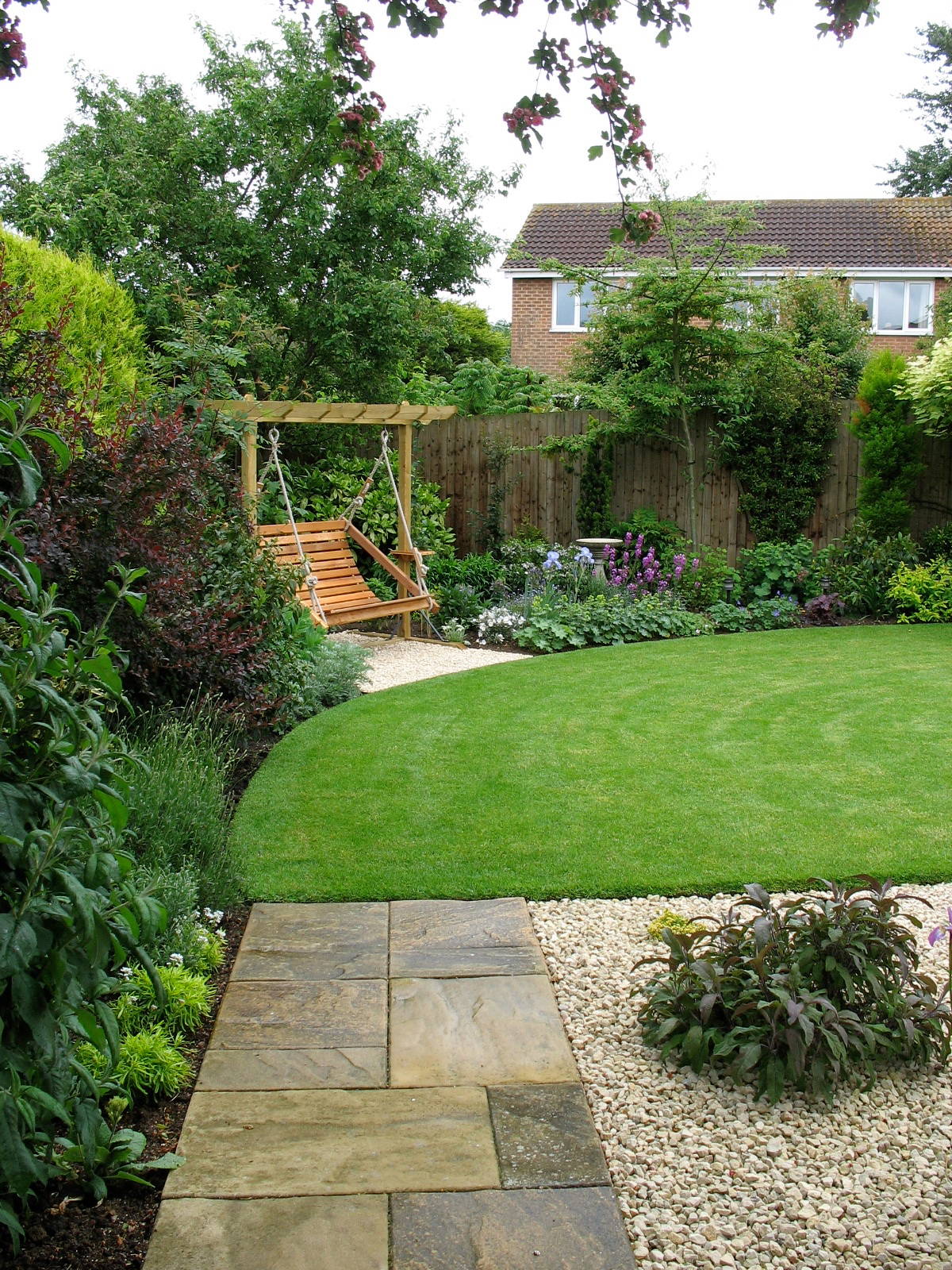A meticulously maintained suburban backyard is showcased in this photograph. Centrally, a light tan cedar pergola stands over a bed of white pebbles, sheltering a wooden swing bench. The yard's green, manicured grass is arranged in a distinct quarter-circle or half-moon shape, complete with circular lawnmower lines suggesting a recent trimming. A paver walkway in light tan and grey hues extends into the scene from the foreground, bordered on the right by an area filled with gravel, landscaped plants, and shrubs, including hostas. Along the left edge of the lawn, the privacy fence is adorned with a variety of blooming perennial flowers, Chinese fringe, monkey grass, and small trees, creating a vibrant display of spring or early summer flora. Purple irises and a birdbath add touches of color and charm, while a towering green tree in full leaf and the backdrop of a modest-sized, two-story brick house beyond the fence underscore the suburban setting. The sky overhead appears white, adding a neutral, serene background to the lush scenery below.